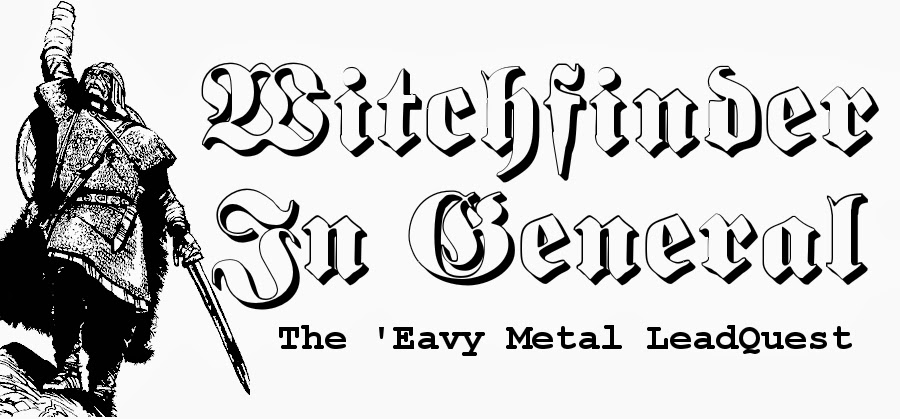The black and white image appears to be a promotional banner, likely for a medieval-themed video game or shop. Dominating the right side, the title "Witchfinder in General" is prominently displayed in an ornate, large, medieval-type font with a shadow effect, making the text appear elevated and striking. Below this, in smaller Courier font, it reads "The Evie Metal Lead Quest," with "Evie" stylized with an apostrophe before the 'E,' omitting the 'H.'

On the left side of the image, there is an intricately drawn character resembling a medieval warrior or knight. The character is clad in armor, including a helmet and a pelt cape. They are depicted standing atop a rocky surface, giving a commanding presence. Their left hand grips a sword pointed downwards, while their right arm, which appears to be raised, ends in a stump as the hand is missing or possibly obscured by the image's edge. A shield is strapped to their back, completing the warrior's formidable appearance. An arm bandage is visible on their raised right arm, adding an element of rugged realism to the artwork.